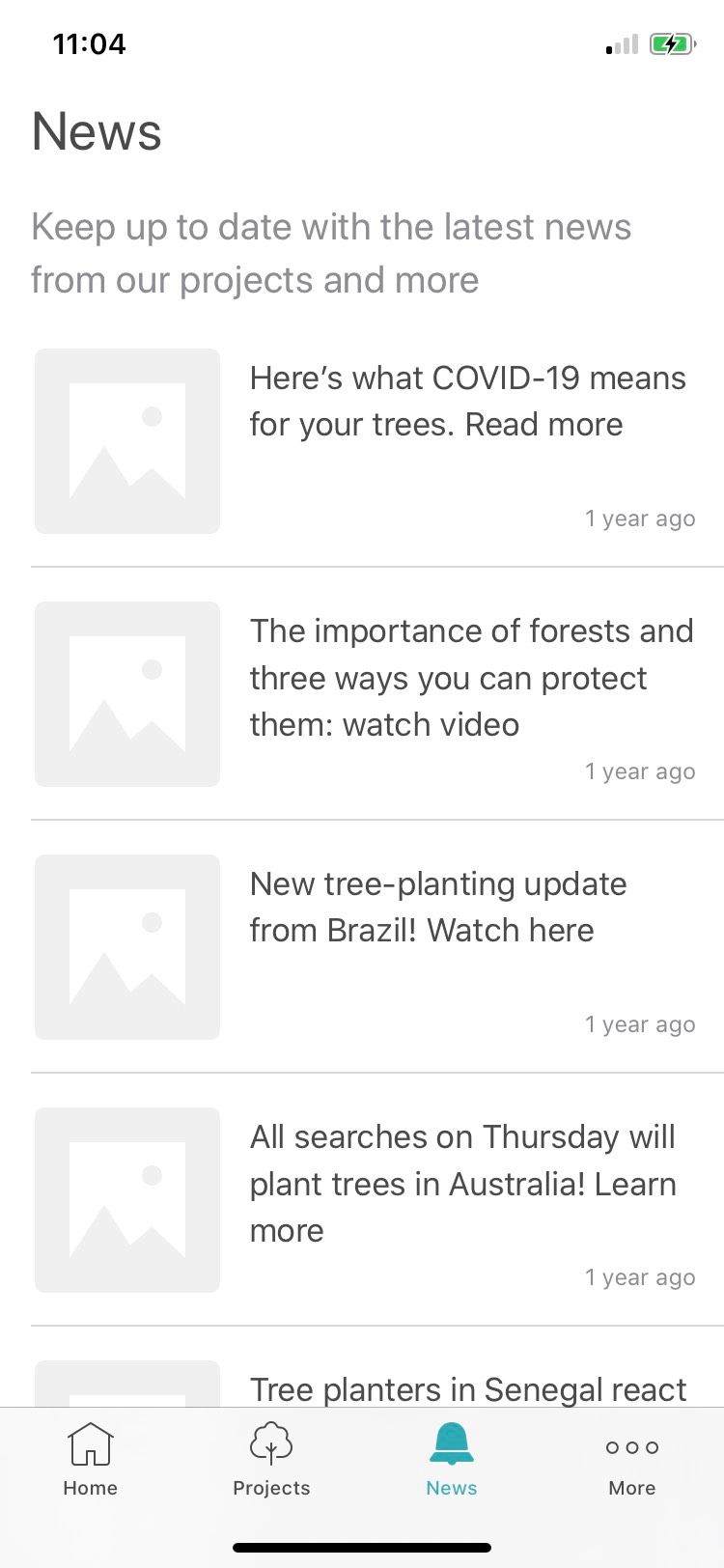This is a detailed screenshot of a cell phone screen. 

- **Top Section of the Screen:**
  - **Left Corner:** The time displayed is 11:04, with no indication of AM or PM.
  - **Right Corner:** Icons are present showing:
    - A battery charging indicator.
    - A cellular signal strength indicator, displaying one out of four bars, signifying a very low signal.

- **News Section:** Below the top bar, in a black font, the word "News" is prominently displayed.
  - Underneath, in gray letters, the text reads: "Keep up to date with the latest news from our projects and more."
  - The subsequent headlines are listed chronologically:
    - **First Headline:** "Here's what COVID-19 means for your trees, read more." This article is noted to be from one year ago.
    - **Second Headline:** "The importance of rainforests and the three ways you can protect them, watch video," also marked as one year old.
    - **Third Headline:** "New tree-planting update from Brazil, watch here," again, from one year ago.
    - **Fourth Headline:** "All searches on Thursday will plant trees in Australia, learn more," from the same time frame, one year ago.
  
Each headline provides a call-to-action either to read more or watch a video, enhancing user engagement with the information on environmental updates and initiatives.